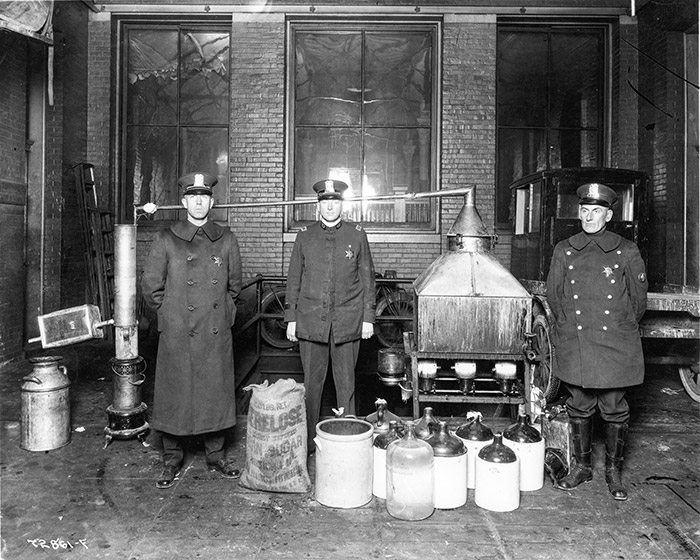This is a black-and-white photograph likely from the 1920s or 1930s, capturing a scene with three policemen standing on a concrete ground in front of a dark, brick building. The building features sections of windows on the left, middle, and right, and a brick wall on each side. The officers, wearing old-timey cop hats and knee-high boots, are dressed in varying styles of overcoats: the left officer in a long, grayish coat, the middle officer in a shorter coat with long sleeves, and the right officer in a coat slightly longer than the middle one, adorned with a lapel and double rows of buttons running diagonally across his chest. 

In the background, a large metal vat is visible, indicating their recent raid on a moonshine operation. Between the left and middle officers, there's a still, and scattered around are various jugs, including white and brown old-timey alcohol containers, and a bag labeled "sugar." Additional elements in the scene include a pile of ten bottles or containers likely containing alcohol, some piping, and an old-style bike leaning against the building. This detailed image vividly depicts a moment in time when the policemen successfully intercepted an illegal moonshine production.